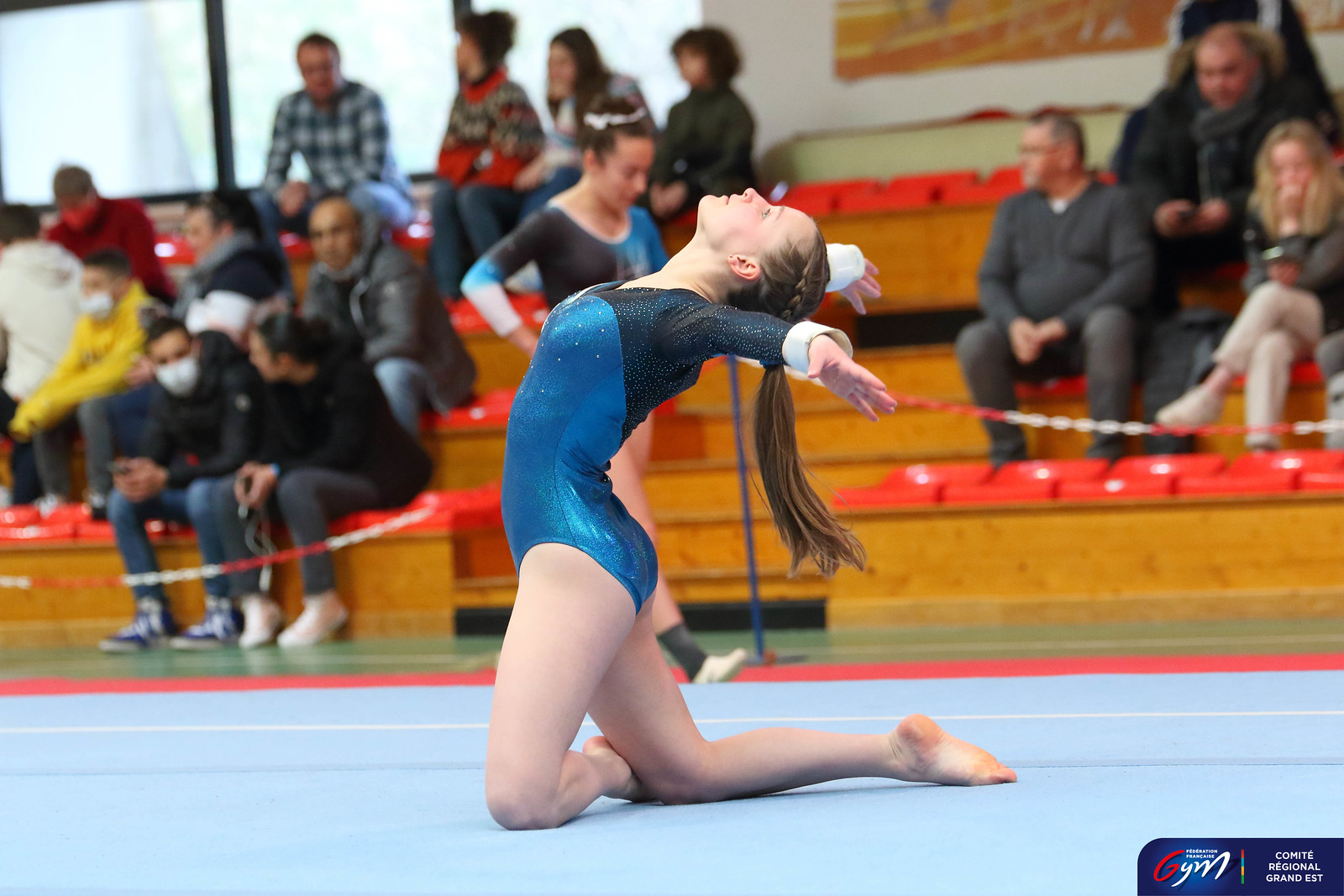In this captivating photograph, a young female gymnast is captured in a dramatic, arched-back pose during a floor exercise. She dominates the foreground, kneeling on a light blue mat with a red border. Her head is tilted back so far that her eyes are gazing at the ceiling, and her hair, gathered in a ponytail, hangs vertically behind her. She is attired in a striking blue leotard with black sleeves and white cuffs, adding a burst of color against the muted background.

The setting appears to be a small gymnasium, suggested by the golden brown-colored bleachers and the variety of spectators in winter coats, implying it's the winter season. The bleachers, which also feature red seats, are sparsely populated, with attendees somewhat scattered and not fully engrossed in the gymnast’s performance.

In the backdrop, slightly blurred to emphasize the main subject, another gymnast can be seen walking towards the right, with her head down and hands on her waist, seemingly preparing for her routine. Large windows in the upper left corner of the image allow some natural light to filter in, adding depth to the composition. The text "Comité Régional Grand Est" is partially visible, indicating the venue's location. The overall color palette includes tones of blue, orange, brown, yellow, red, white, and black, weaving together to create a vivid and dynamic scene.